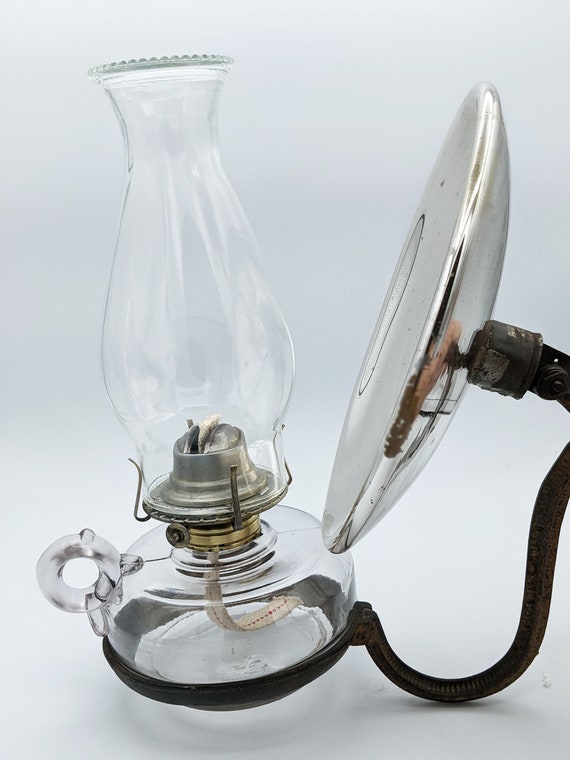The image showcases a close-up view of a vintage oil lamp, prominently featuring its intricate design elements. The lamp has a transparent glass covering, revealing the internal burner, which appears to be made of stainless steel. Notably, the oil reservoir at the bottom of the lamp is empty and shaped like a glass bowl. There is no top tube, just the flared opening where smoke would normally escape.

On the left side of the lamp is a visible loop, while the entire structure is supported by a round cradle at the bottom. To the right of the lamp, a metallic, bulbous apparatus is seen, possibly part of a bending mechanism, which is connected to the lamp. Adjacent to this apparatus and slightly behind the lamp, there is a large, dim light fixture that appears to be off or unplugged. The entire scene is set against a gray-colored background, highlighting the details and vintage appeal of the lamp.